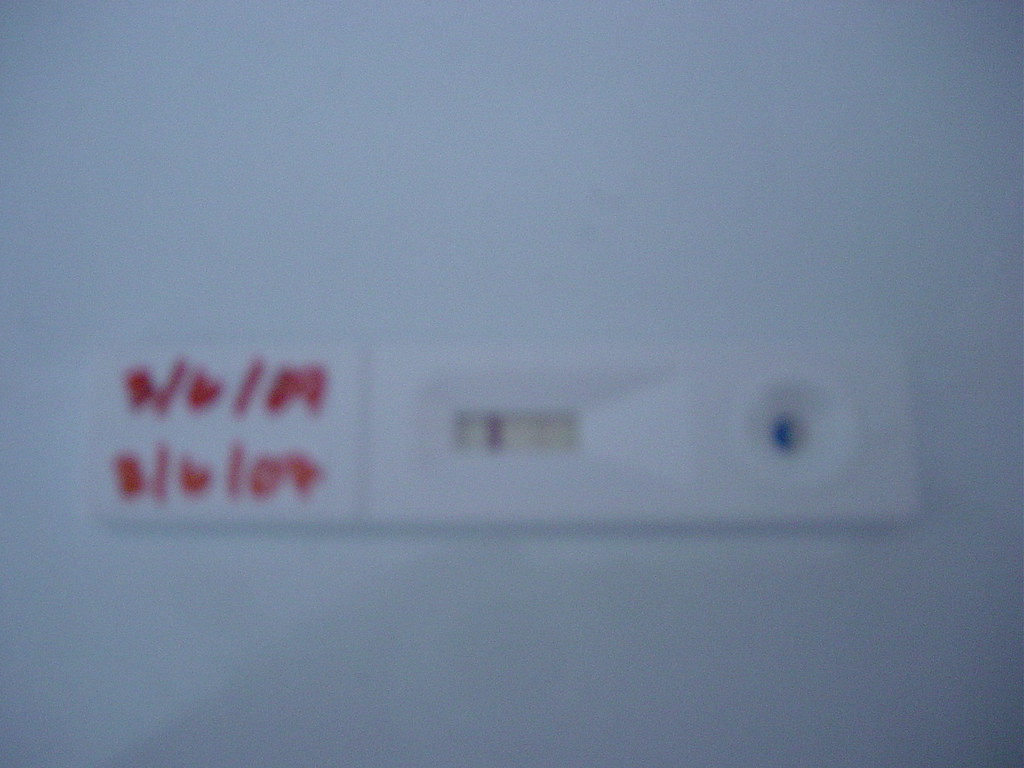A slightly blurry image features a solitary rectangular object positioned slightly downwards from the center against a solid white background. The object displays red inscriptions on the left side: "S/V/M" on the top left half and "S/V/OV" on the bottom left half. These sections are separated by a vertical line. The middle portion of the object contains a smaller rectangular area with a see-through, tan-colored background intersected by a vertical solid black rectangle. On the far right, the object includes a circular component, within which a smaller circle holds a dark blue crescent-shaped moon.